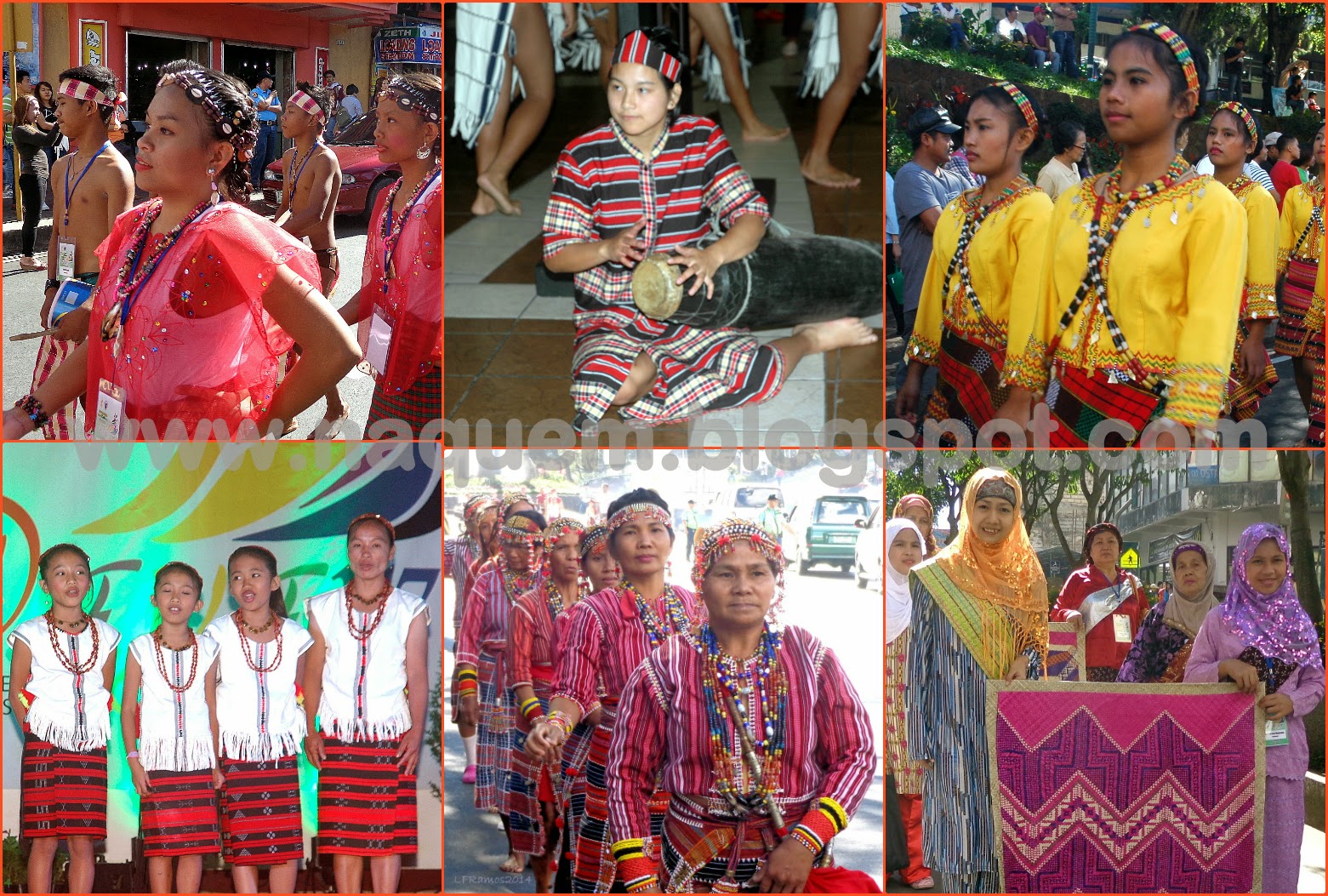This vibrant composite image consists of six photos showcasing people, mostly women and girls, possibly from an ethnic Asian background, engaging in various cultural activities, possibly in Malaysia or the Philippines due to the presence of hijabs. The top left photo depicts a parade under a sunny sky, with a young girl marching among other participants. In the center top image, a young boy energetically plays a drum. The top right image features three girls adorned in yellow long-sleeved shirts, beaded hair, and matching red and black skirts. At the bottom left, several girls are dressed in white sleeveless tank tops with frilly bottoms and red and black striped skirts, mirroring the attire of those in the top right image. The middle bottom image shows older women in pink and purple striped long-sleeved shirts walking in a straight line, while the bottom right photo captures women wearing hijabs, possibly holding quilt work over their heads. A website watermark, "www.naquem.blogspot.com," is visible in the middle of the composite.